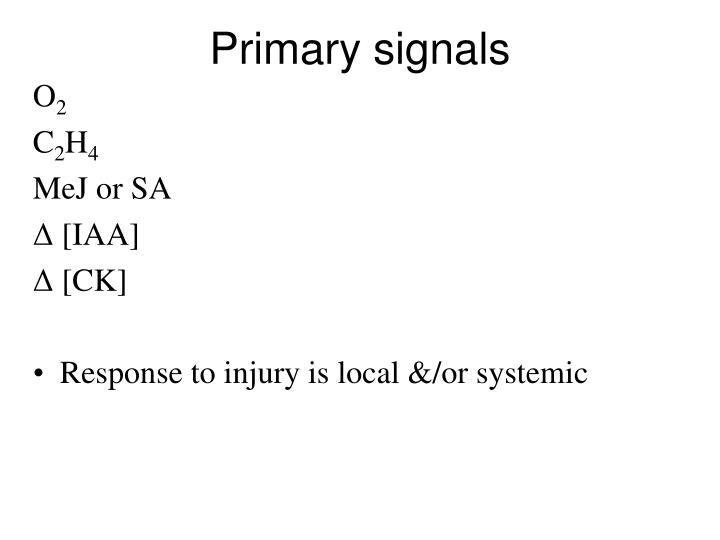The image depicts a white background featuring black text and symbols. At the top center, it reads "Primary Signals" in bold black font. Below, aligned to the left, there is a sequence of chemical symbols and acronyms starting with "O₂," followed by "C₂H₄," and "MEJ or SA." Further down, there are two triangle symbols, the first labeled with "IAA" inside parentheses and the second with "CK" in parentheses. At the bottom left, a bullet point notes, "response to injury is local and/or systemic." The arrangement of text is well-spaced, resembling a slide from a scientific PowerPoint presentation likely intended for a classroom setting, specifically in a biology or chemistry context.